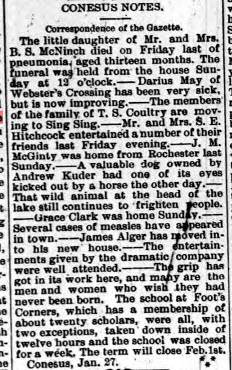The black-and-white image is an old newspaper clipping titled "Canesis Notes, Correspondence of the Gazette." It details various events and updates from the local town. The primary focus is on the unfortunate death of the 13-month-old daughter of Mr. and Mrs. B.S. McNinch, who passed away last Friday from pneumonia, with her funeral held from the house on Sunday at 12 o'clock. The clipping also notes that Darius May of Webster's Crossing has been very sick but is currently improving. Other updates include the family of T.S. Coultry moving to Sing Sing, Mr. and Mrs. S.E. Hitchcock hosting friends last Friday evening, and J.M. McGinchty being home from Rochester last Sunday. An incident involving Andrew Cooter's dog losing an eye after being kicked by a horse is mentioned, along with reports of a wild animal at the head of the lake causing fright among the townspeople. Additional news includes several cases of measles in town, James Auger moving into his new house, and the well-attended entertainments by the Dramatic Company. The report also mentions the spread of "the grip," a term likely referring to influenza, affecting many residents and leading to the temporary closure of a school at Foote's Corners. The term for the school is set to close on February 1st, with Finesse January 27.